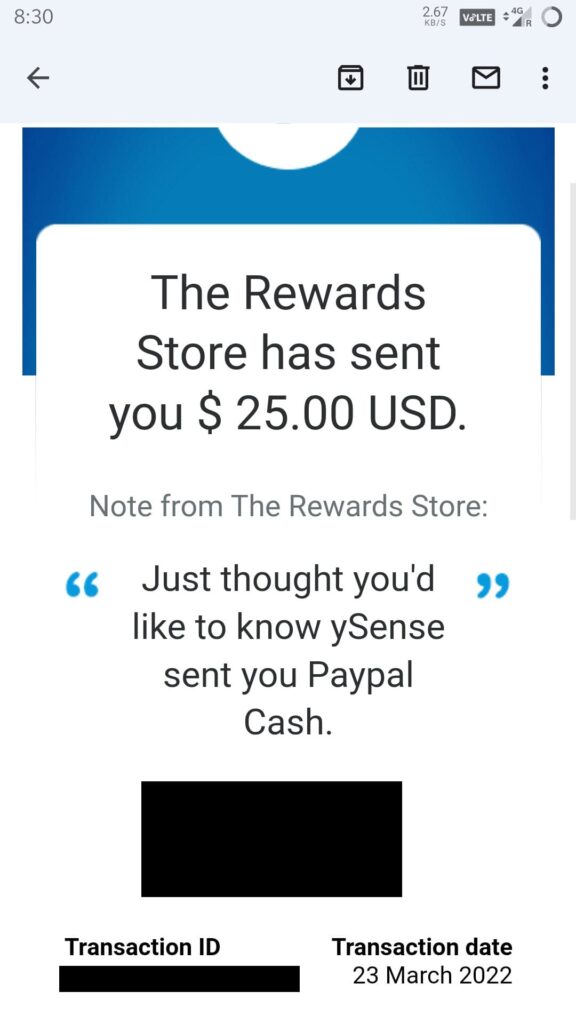This is a detailed screenshot of a notification from a reward store. The screenshot is divided into two main sections: a blue header at the top and a white section below.

In the white section, the text is primarily focused on informing the recipient about a reward. At the top of this section, bold black text reads: "The reward store has sent you $25 USD." Underneath this, in smaller gray text, it states: "Note from the reward store."

Below this note, a message highlighted in blue reads: "Just thought you'd like to know why sent you PayPal cash." 

Further down, a black rectangle obscures sensitive information, likely for privacy purposes. Below this blacked-out portion, there are two pieces of information: on the left, the "Transaction ID," which is hidden by a black mark, and on the right, the "Transaction date," which is specified as "23 March, 2022."

This cleaned and detailed description should provide a clear understanding of the screenshot content.